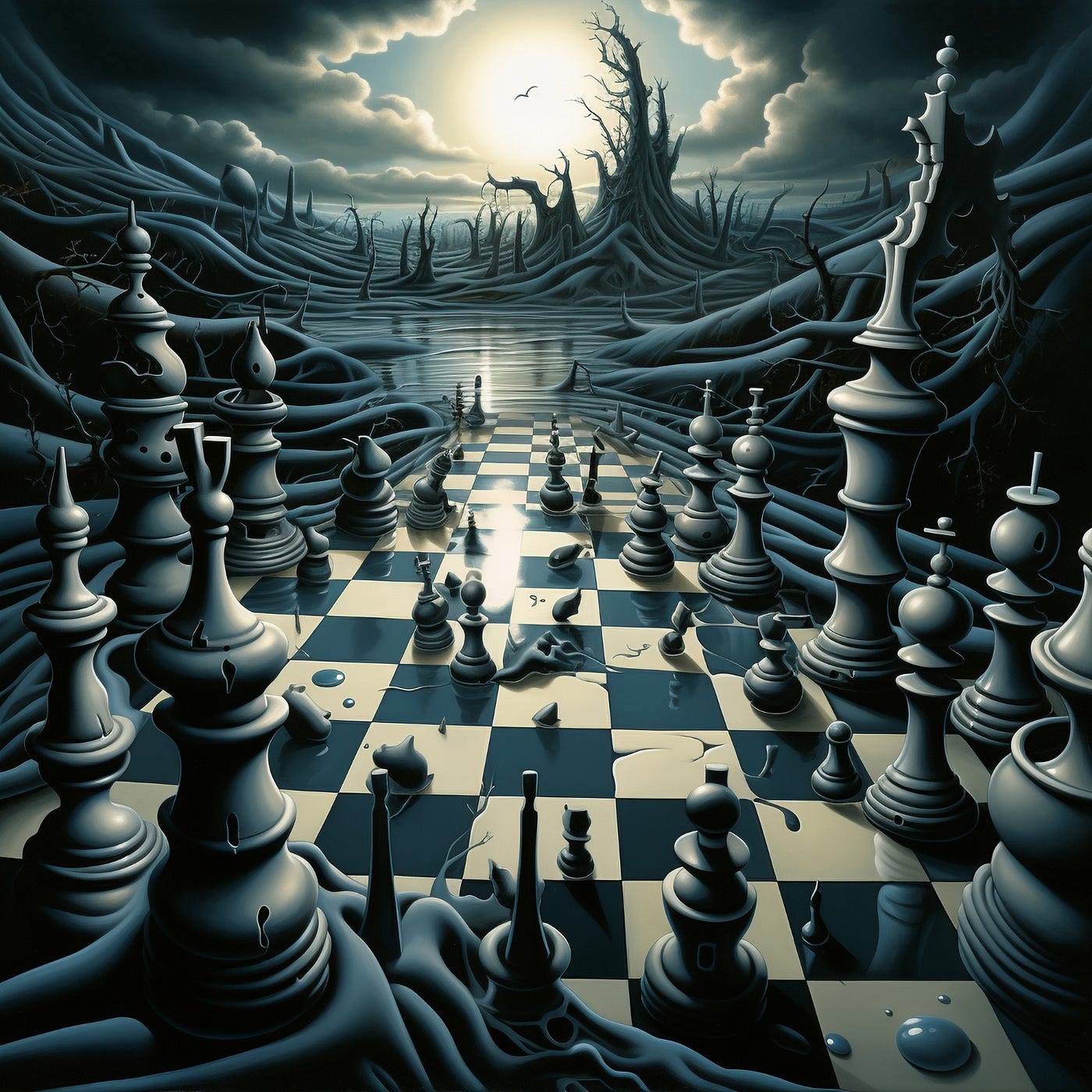This AI-generated image captures an eerie, gothic scene with an intricate interplay of surreal elements. Dominating the foreground is a tan and black checkerboard chessboard that descends into a murky, oily lake, appearing as though some pieces are melting and distorting in a nightmarish fashion. Creepy, twisted branches frame the imagery like wavy black lines, adding to the ominous feel. In the background, the sun sits at the top center, framed perfectly by scraggly trees, with a single bird silhouetted against it. Clouds part just enough to let the sun shine through, casting a haunting reflection onto the water. The entire palette is an unsettling blend of black, white, and gray, amplifying the image's overall atmosphere of dread.